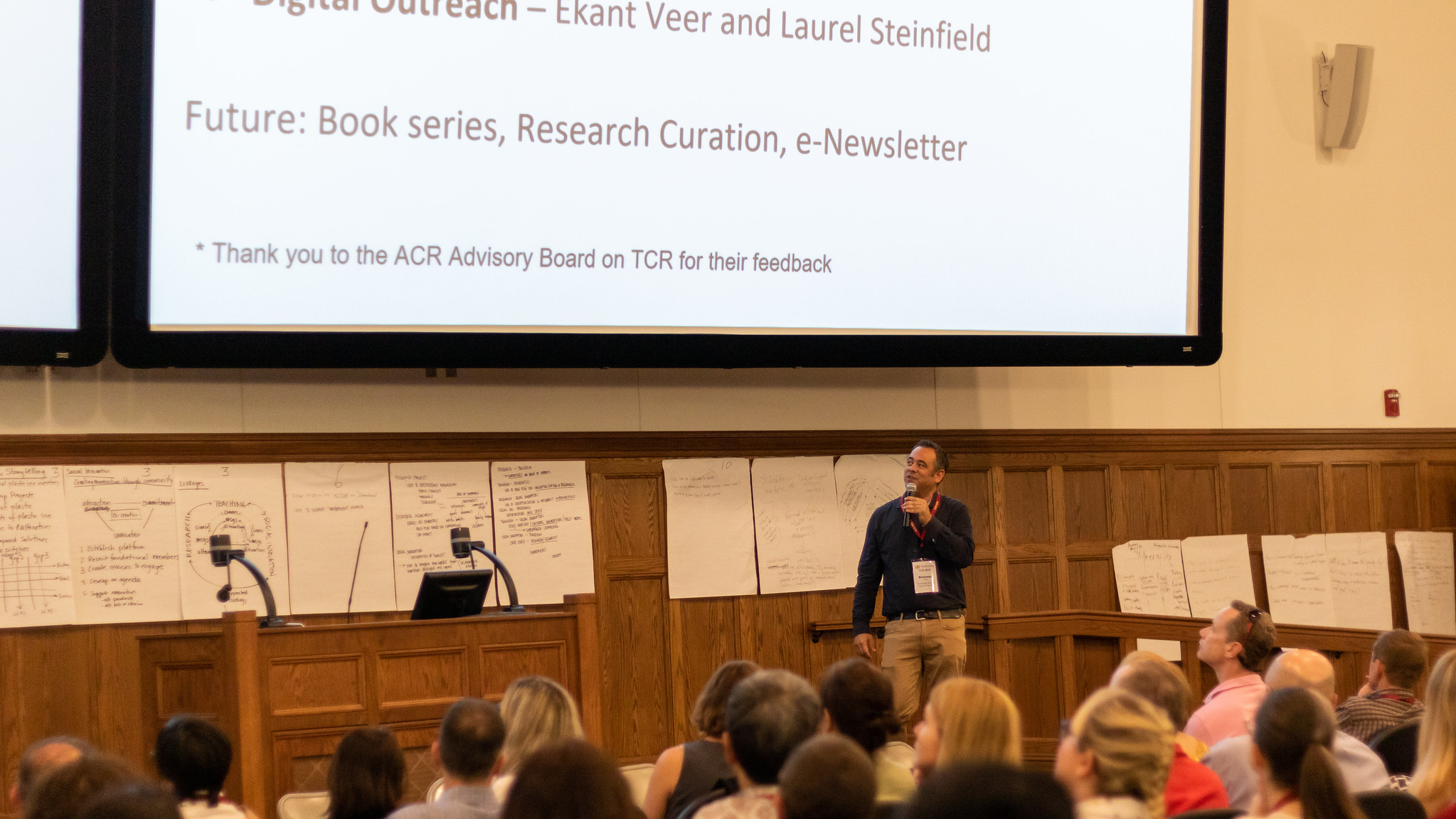The photograph captures a man delivering a lecture in a large classroom or lecture hall. He stands to the right of a podium equipped with a computer, addressing an audience with the aid of a microphone. The man, dressed in khaki pants and a blue button-down shirt, has a lanyard with a badge around his neck. He gazes upward at a series of screens behind him, which display partial text: "future book series," "research curation," and "e-newsletter," followed by, "thank you to the ACR Advisory Board and TCR for their feedback." The backdrop consists of wooden square paneling adorned with various large pieces of paper containing notes and diagrams. The audience, seated and attentively watching, includes both men and women who also look up at the screens.